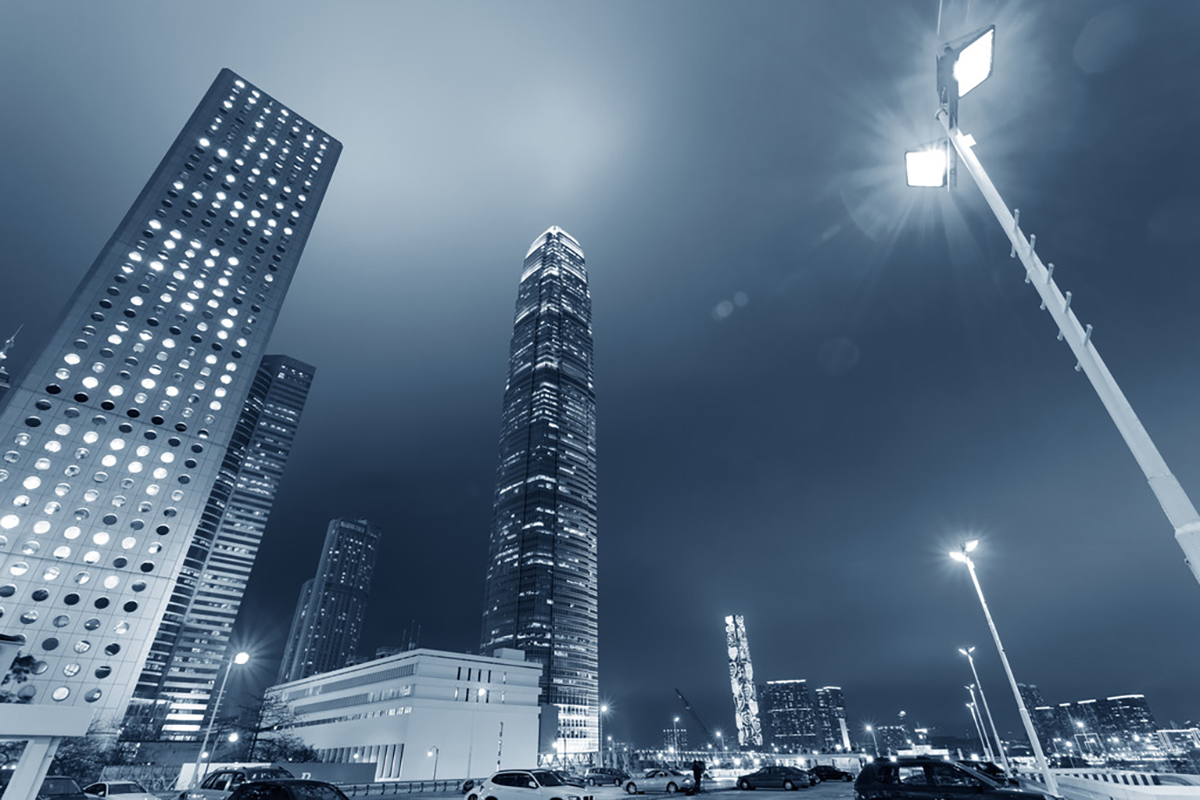An evocative black-and-white nighttime photograph captures the towering presence of five high-rise buildings dominating the left half of the frame, their windows aglow with light. The tallest skyscraper, both distant and strikingly bright, tapers into the background of the image, emphasizing the depth and scope of the urban landscape. Dotted with streetlights that cast an ethereal glow upwards, the scene is tinted in hues of dark blue, white, and various shades of gray. The right half of the image features a parking lot and a walkway where partially visible figures move under the streetlights. The grounded perspective suggests the photo was taken from a low angle, emphasizing the towering nature of the buildings while capturing the intricate details of parked cars, lit streetlamps with metal prongs, and the serene ambiance of a city at night.